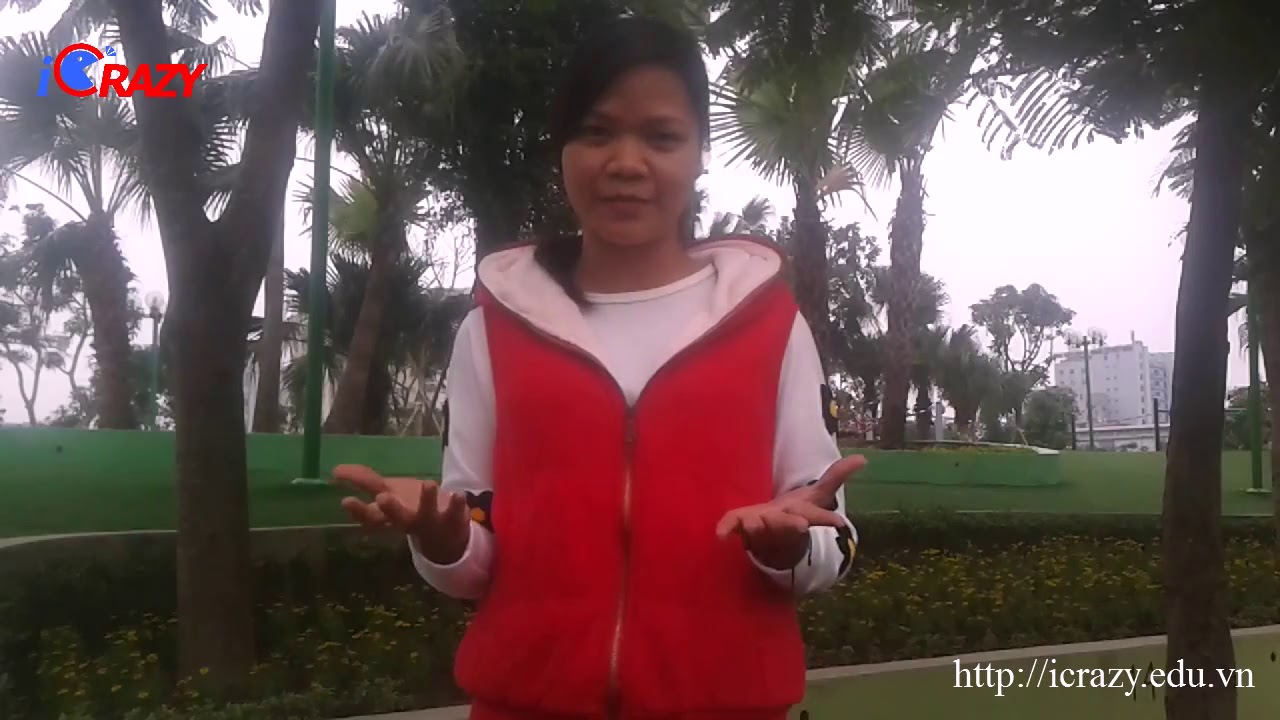In this photo, a woman who appears to be of Southeast Asian or Hawaiian descent, possibly in her early 40s, stands outdoors with a lush background of green grass and numerous palm trees. She has dark brown skin and black hair styled in a ponytail that drapes over one of her shoulders. She wears a red hooded vest over a white long-sleeve shirt. Her hands are extended in front of her with her palms open, suggesting a gesture of explanation or presentation. The photo is taken in what appears to be a park or landscaped area, featuring some flowers, a small stone wall, and scattered light poles. In the mid-right background, there is a white building. The image includes a logo in the top left corner that reads "iCrazy" with the "I" in blue and "crazy" in red. In the bottom right corner, the website address "http://icrazy.edu.vn" is clearly visible in white text.